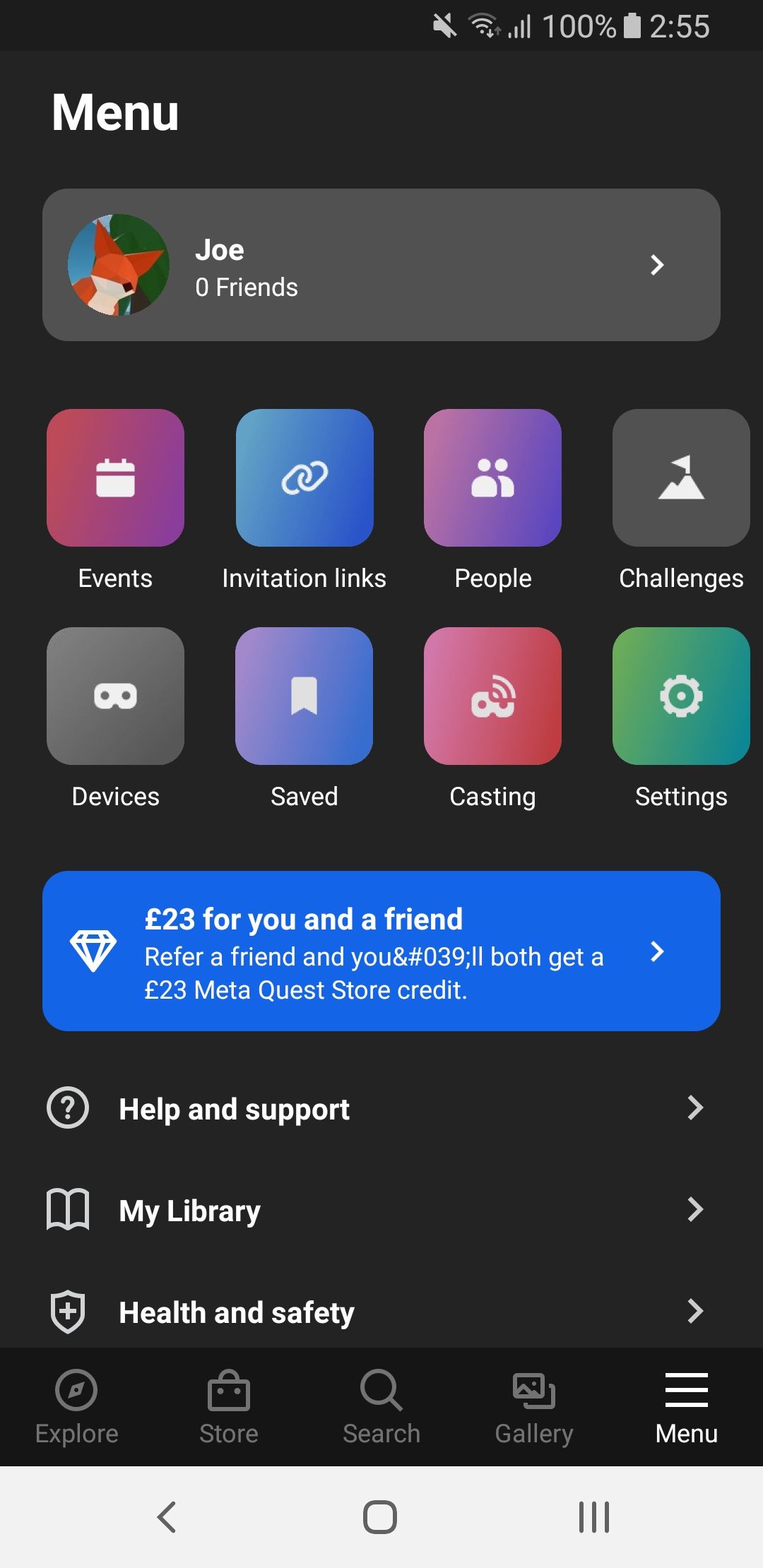The image, set against a stark black background, is a detailed screenshot from a cellphone interface. In the upper right corner of the screen, there are several status indicators: a notification stating "Notifications off," followed by icons showing a strong Wi-Fi connection, a fully charged battery at 100%, and the current time displayed as 2:55.

Dominating the upper left of the display is the word "Menu" in large, bold white letters. Directly underneath, the user, identified as "Joe," has zero friends. Joe’s profile picture is a charming, cartoon-like illustration of a fox encapsulated in a circular frame.

Further down the screen, there are organized rows of menu options. The first row contains four boxes labeled "Events," "Invitation Links," "People," and "Challenges." The subsequent row showcases another set of menu options: "Devices," "Saved," "Casting," and "Settings."

Towards the bottom of the screen, there is a prominent blue box containing text alongside a white diamond logo. The text states, "£23 for you and a friend," suggesting a potential promotional offer.